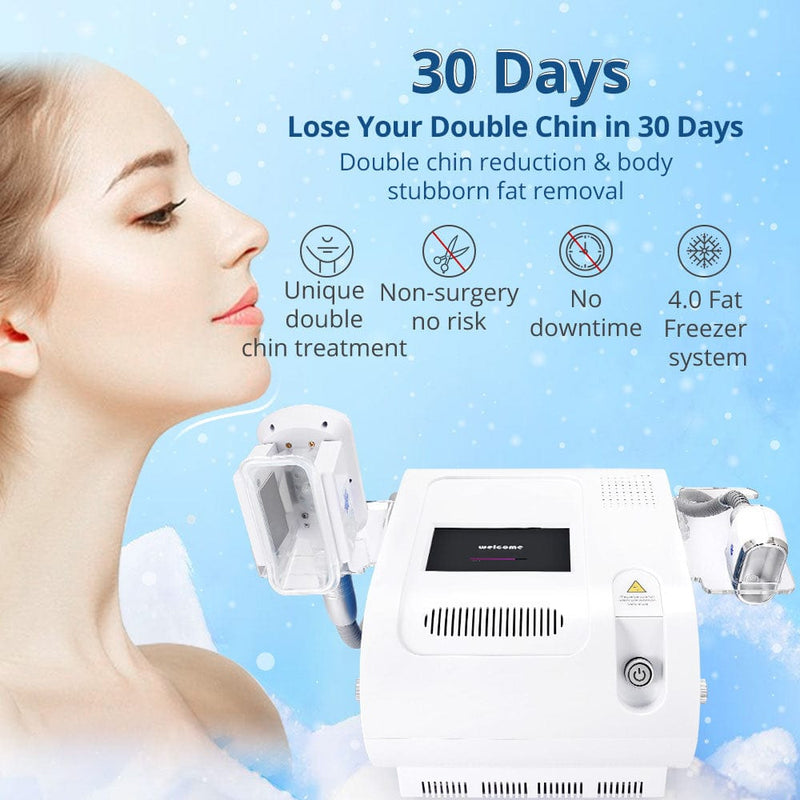This advertisement features a product designed for double chin reduction and stubborn body fat removal. The backdrop is a gradient blue, lighter at the top left and transitioning to a darker blue, creating a clean and enticing visual. Dominating the left side of the image is the side profile of a smiling, beautiful woman with a long neck and pink lipstick, highlighting her chin and neck area. 

To the right bottom corner, there's a photograph of the product: a white, rectangular machine with attached accessories, a black rectangular top, several vents, and a power button. Above the woman, bold blue text prominently states, "30 days to lose your double chin," accompanied by additional promises like "double chin reduction" and "body stubborn fat removal."

Further emphasizing the product's benefits, four circular logos are arranged vertically beside the machine. The logos declare "unique double chin treatment," "non-surgery," "no risk," "no downtime," and "4.0 fat freezer system." The illustration at the top, in grey, ties the design elements together, ensuring the advertisement is cohesive and informative.